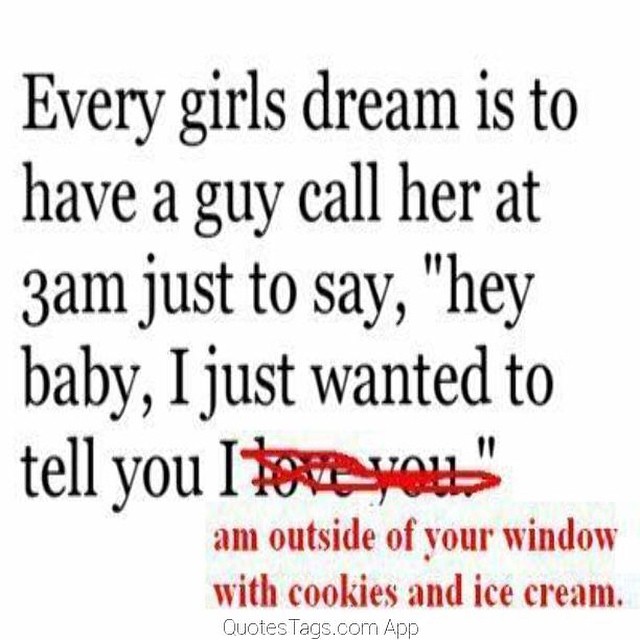The image features a quote in predominantly black text against a white background. It reads: "Every girl's dream is to have a guy call her at 3 a.m. just to say, 'Hey baby, I just wanted to tell you I love you.'" The phrase "I love you" is crossed out in red pen. Below this, in smaller red text, it continues with, "I am outside of your window with cookies and ice cream." At the bottom center of the image, in a light gray serif font, the text "quotes.tags.com app" is displayed. The overall design includes a blend of different fonts and text sizes to emphasize various parts of the quote.